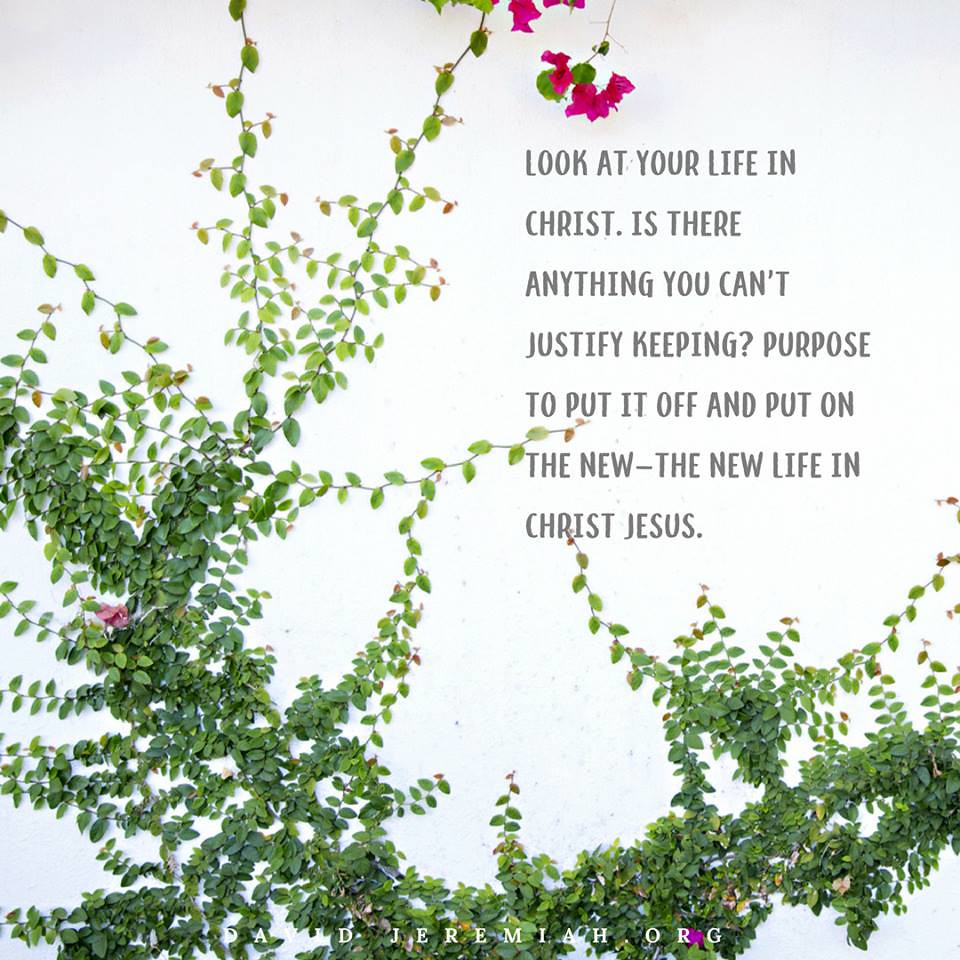The square photograph features an elegant arrangement of green leaves on a predominantly pale white background that subtly transitions to a light blue hue at the bottom. The leaves, resembling ivy, are densest in the lower left corner and gracefully arc around, fanning out towards the right and up. Scattered among the leaves are a few purple petals, with a larger cluster of magenta-colored flowers emerging from near the top center. These flowers, attached to thin green stems, are accompanied by green leaves. Underneath this floral arrangement, bold gray text reads, "Look at your life in Christ. Is there anything you can't justify keeping? Purpose to put it off and put on the new. The new life in Christ Jesus." At the very bottom of the image, against the green backdrop of the ivy, white text states "davidjeremiah.org."